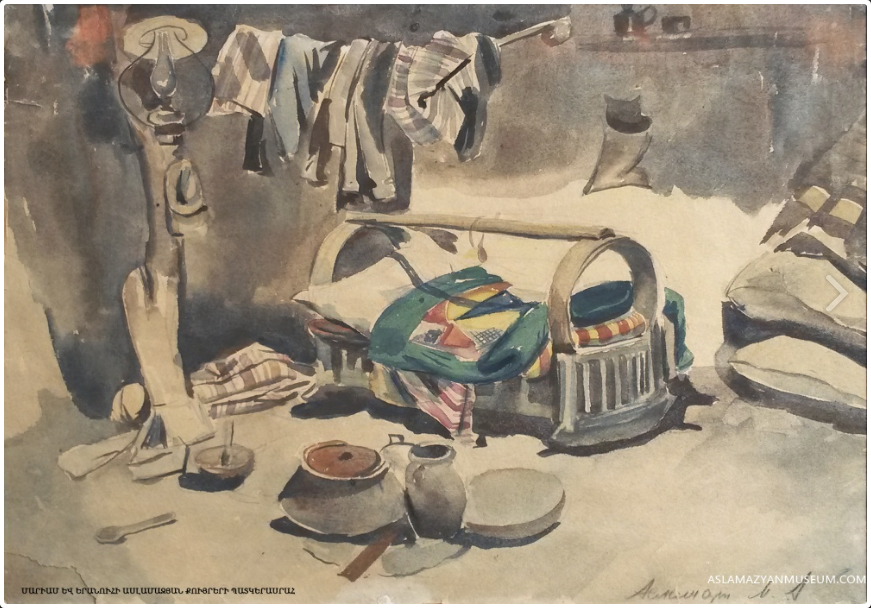This painting, rendered in acrylic, depicts the interior of a modest and dilapidated room, likely belonging to a poor individual. Dominantly shown is a makeshift baby bed with a green blanket, complemented by a yellow and red mattress and a pillow. The bed’s structure appears to be rudimentary, possibly constructed from rock, which mirrors the rocky texture of the room’s walls and surfaces. Above the bed, a row of clothes hangs draped over a long pole, further emphasizing the austere living conditions. Scattered on the floor are various utensils, including a pot, a plate, a bowl, a jug, a cooking whistle, and spoons, adding to the sense of daily life in a humble setting. A night lamp is also seen hanging from a pole. The painting primarily features a black and white palette with occasional splashes of color, enhancing its modernist and somewhat abstract feel. The background wall appears unpainted and in poor condition. Notably, the bottom right corner bears the artist's partially legible signature starting with 'A', alongside the website AslamMaziMuseum.com, written in white font just above.